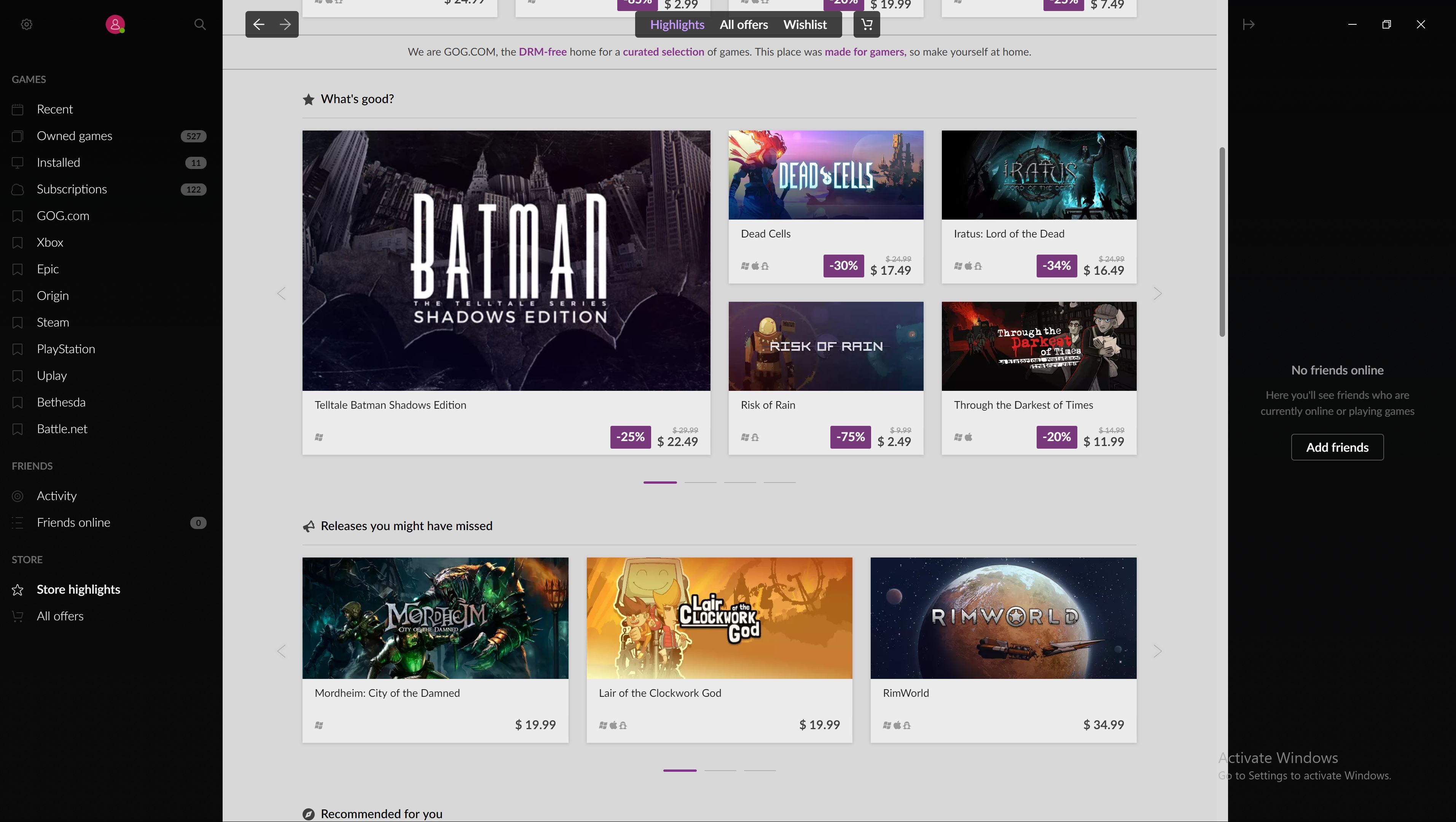The image displays an online gaming platform interface with a dark-themed, black background on the left sidebar and white text for menu options. At the top of this sidebar, there are three icons: a settings icon, a pink profile icon, and a search icon. Below these icons, the text reads "Games," followed by categories such as "Recent Owned Games," and lists indicating 27 installed games and 11 subscriptions. Various gaming platforms are also listed, including GOG.com, Xbox, Epic, Origin, Steam, PlayStation, Uplay, Bethesda, and Battle.net.

Further down the sidebar, there are sections labeled "Friends," "Activity," and "Friends Online (0)." The "Store" section is divided into "Store Highlights," "Store," and "All Offers." The "Store Highlights" option is currently selected, indicated by its text being whiter than the other menu items.

In the center of the image, there is a main content area with three tabs: "Highlights," "All Offers," and "Wishlist." The "Highlights" tab is active and highlighted in purple. Beneath this tab, a welcome message reads, "We are GOG.com, the DRM-free home for a curated selection of games. This place was made for gamers, so make yourself at home." Below the message, several game titles and their prices are listed:

- Batman Telltale Series - Batman Shadows Edition: $22.49
- Dead Cells: $17.49
- Iratus: Lord of the Dead - $16.49
- Through the Darkest of Times - $11.99
- Risk of Rain - $2.49
- Mordheim: City of the Damned - $19.99
- Lair of the Clockwork God - $19.99
- Rimworld - $34.99

The prices are shown in black text, and the game covers and titles are arranged neatly in the content area.